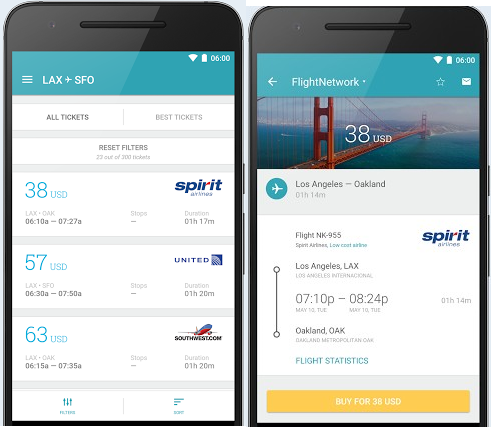The image features two black mobile devices displaying flight booking applications. The screen of the device on the left shows a flight search interface with a teal blue navigation bar at the top. It lists flights from LAX to SFO, with options for "All Tickets" and "Best Tickets," as well as a "Reset Filters" button. Displayed flights include Spirit Airlines for $38, United for $57, and Southwest for $63.

The screen of the device on the right is titled "Flight Network," with icons for favoriting and mail in the top left corner of the teal blue bar. Below this, an image of the Golden Gate Bridge is visible. The flight details show a route from Los Angeles to Oakland, operated by Spirit Airlines, with a departure time of 7:10 and an arrival time of 8:24. A "Buy Now" button shows the price of $38 USD.